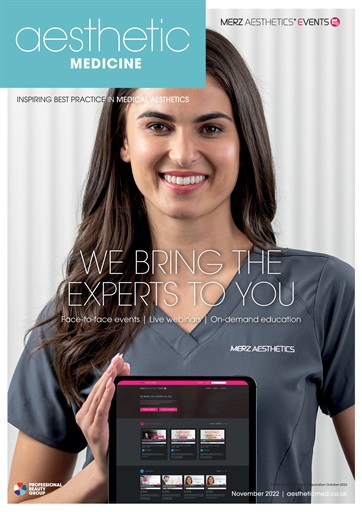The magazine cover features an image of a woman wearing dark grey short-sleeved scrubs, prominently holding up a tablet that displays a website with a pink header and a dark grey body adorned with various tiles and photographs. In the upper left corner of the cover, a light teal blue banner spans about three-fifths of the top, emblazoned with the word "AESTHETIC" in white text, and "MEDICINE" in capitalized, bold sans-serif font. In the top right, the text "MERS AESTHETICS EVENTS" appears, with "MERS" and "EVENTS" in bold grey text, except for the letter 'E' in pink, and "AESTHETICS" in thinner grey text. Adjacent to this is a pink badge featuring a white icon. 

Below the teal header, the phrase "INSPIRING BEST PRACTICE IN MEDICAL AESTHETICS" is prominently displayed, with "IN MEDICAL AESTHETICS" written in white on a teal background, and "INSPIRING BEST PRACTICE" in grey on a white background. Centrally located on the page, large white text in all caps reads, "WE BRING THE EXPERTS TO YOU." Beneath this, smaller white text details three types of educational offerings: "FACE TO FACE EVENTS," "LIVE WEBINARS," and "ON DEMAND EDUCATION," separated by vertical white lines.